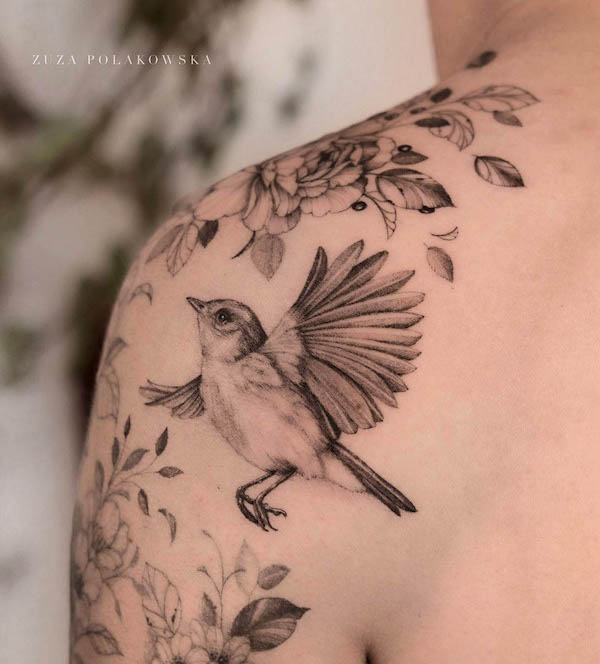This close-up photograph captures a detailed tattoo on the left shoulder and upper arm of an individual, possibly female. The realistic black ink tattoo centers around a small, round bird in flight, its wings prominently spread and its feet tucked slightly as if mid-landing. Intricately rendered, the bird is surrounded by an ornate floral design featuring roses, leaves, and small berries. The floral elements wrap around towards the front of the shoulder and extend down the arm, suggesting a natural habitat for the bird. The tattoo artist's name, "Zuza Polakowska," is inscribed at the top left-hand corner of the image. The backdrop is a blurred outdoor setting, emphasizing the intricate artwork on the subject's shoulder.